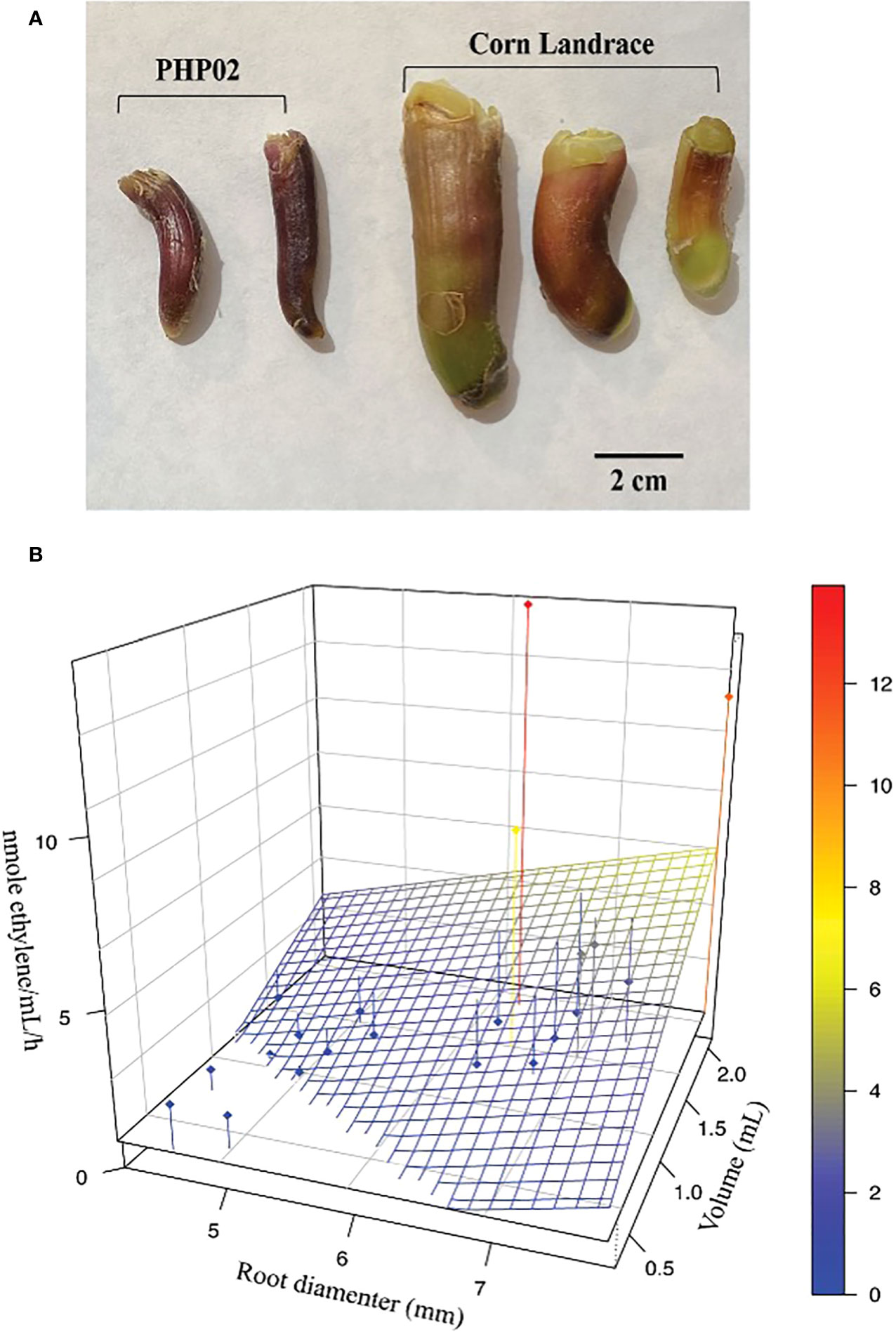The image comprises two distinct visuals. Visual A is a photograph displaying five items that closely resemble shriveled fingers or roots. The two items on the left are smaller, more shriveled, and darker in color, labeled "PHP 02." The three items on the right are plumper, slightly green, and labeled "Corn Landrace." Visual B is a graph located beneath the photograph, which measures the root diameter in millimeters and the n-mole ethylene per milliliter per hour. The graph also includes a volume measurement in milliliters. It features a diagonal blue and yellow line and a colorful scale on the right ranging from 0 to 12, transitioning from blue through yellow, orange, and red, possibly indicating temperature changes or another varying parameter.